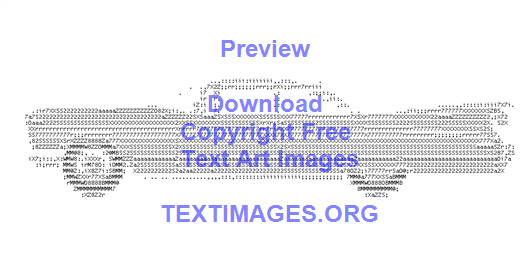This image showcases a detailed grayscale clipart of a vintage 1950s or 1960s Chevrolet-style automobile. The car exhibits classic features such as a long front engine, an elongated rear trunk with distinctive fins, and dark gray tires. Overlaying the car is a light purple text that states, "preview. Download copyright-free text art images, textimages.org." The background is white, and the car is composed of random text characters, creating an ASCII art representation.